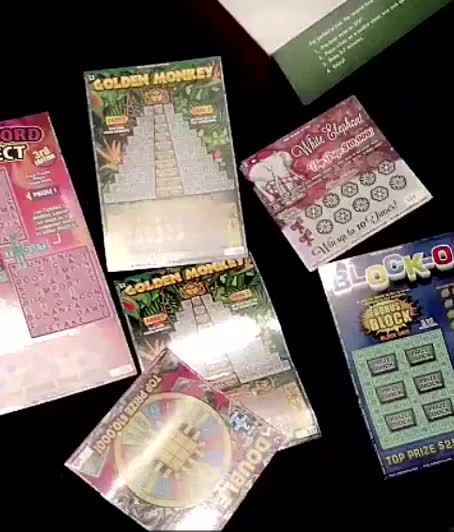The photograph showcases a collection of six unscratched lottery tickets spread across a table with a solid black background. On the left side, the edge of a large, bright pink ticket is visible, with partial text showing "ORD" and "CT," along with a circular area labeled "THIRD." In the center-left, two identical rectangular tickets with a jungle theme read "GOLDEN MONKEY" in bold yellow letters, featuring an illustration reminiscent of a pyramid. Directly below one of the Golden Monkey tickets is a square-shaped card that reads "DOUBLE" and depicts a large wheel, advertising a top prize of $10,000. In the upper right corner, a square ticket titled "WHITE ELEPHANT" features an image of a white elephant with snowflakes. Below that, a blue rectangular ticket labeled "BLOCKO" depicts blocks and includes a scratchable area. The detailed arrangement and variety of the tickets imply they were recently purchased, potentially holding unclaimed prizes.